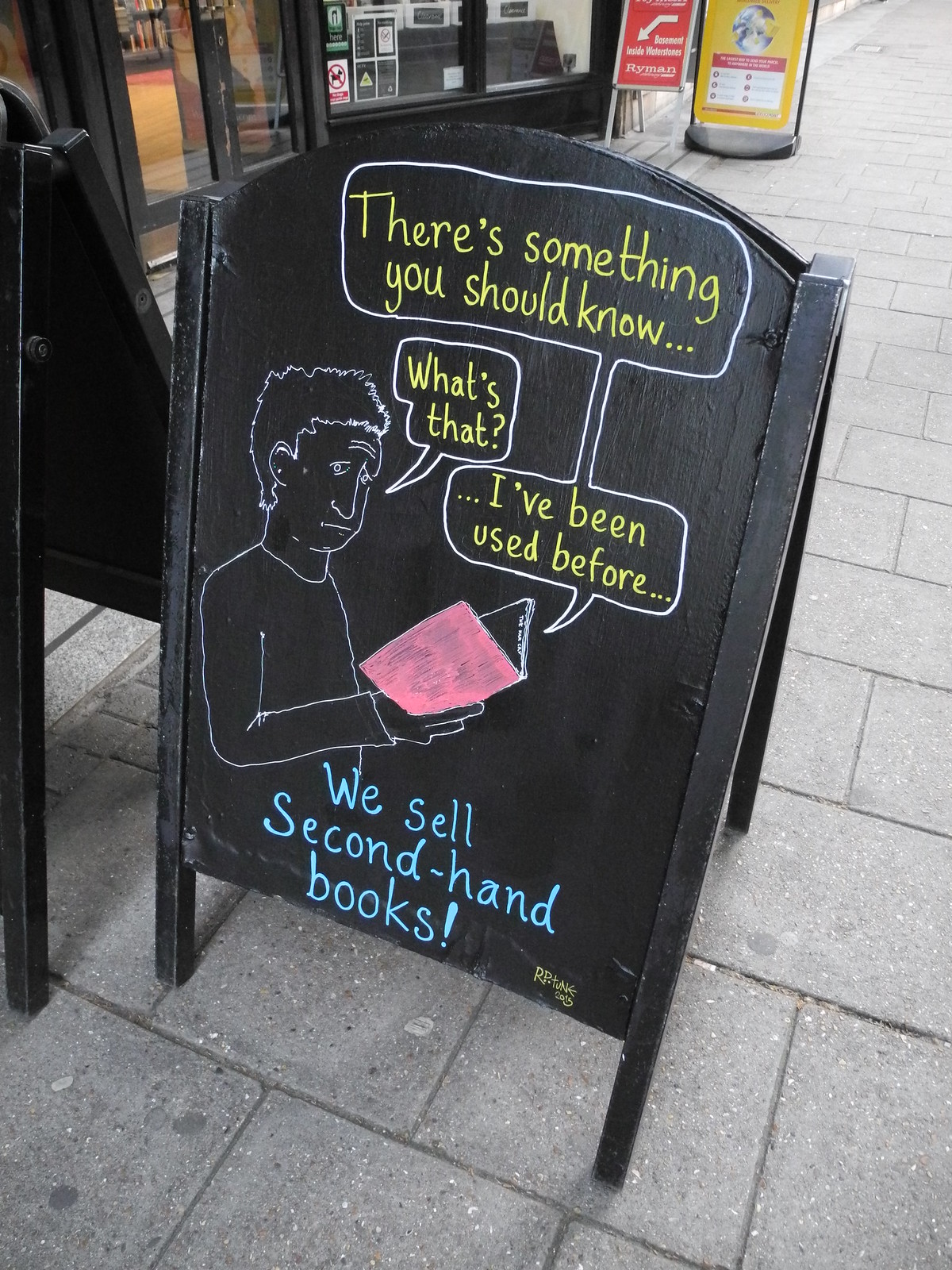The photograph shows a black-painted wooden sign positioned on a grey stone-bricked sidewalk outside a second-hand bookstore. The sign is centrally placed in the image and depicts a chalk drawing of a man with a somber expression, looking down at an open book with a pink cover. Both the man and the book have white speech bubbles with yellow text. The conversation is as follows: the book says, "There’s something you should know," to which the man responds, "What’s that?" The book replies, "I’ve been used before..." Below this dialogue, written in blue chalk, the sign reads, "We sell second-hand books!" The scene is outdoor, likely set in the middle of the day in an urban environment. The overall color palette includes grey, black, light blue, yellow, red, orange, and pink.